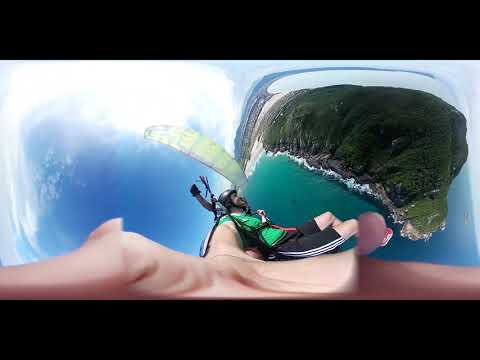The image captures a thrilling scene of a man paragliding above a possibly Hawaiian island, with a breathtaking aerial view taken from what seems to be a GoPro camera, indicated by the fisheye distortion. The paragliding man wears a green shirt, black Adidas shorts with white stripes, and red shoes, and is secured by a harness and helmet. His outstretched arm holds the camera, giving a direct view down his arm. Above him, a light lime-green parachute hints at a tandem flight, with another person’s hands visible, holding the directional pull strings. The scene unfolds under a bright daytime sky, mostly blue with scattered white clouds. Below, a stunning blue-green ocean with crashing waves meets the rugged shoreline of a lush, mountainous island adorned with green trees. The image is further framed by thick black borders on the top and bottom, emphasizing the incredible height from which this magnificent landscape is observed.